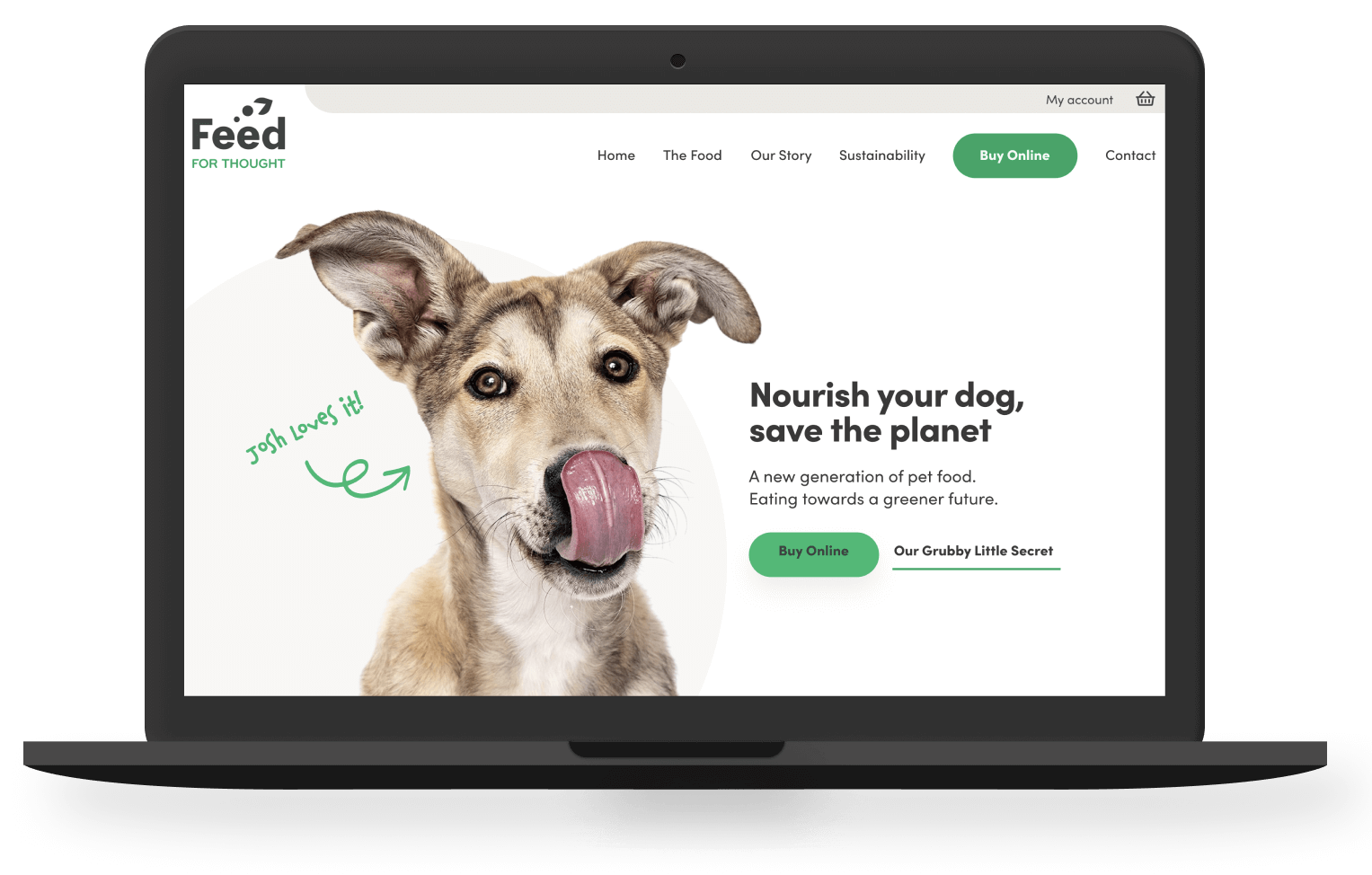A detailed screenshot of a laptop displaying a webpage for a pet food company. At the top left, the site features the logo "Feed for Thought." The navigation menu below includes sections labeled "Home," "The Food," "Our Story," and "Sustainability," followed by a prominent green "Buy Online" button and a "Contact" link. The main banner headline reads, "Nourish your dog, save the planet," with a subheading, "A new generation of pet food, eating towards a greater future." Below, another green "Buy Online" button is prominently placed. On the right side, a caption titled "Our grubby little secret" is displayed. To the left, there's a picture of a dog licking its nose, highlighted by a spiral arrow pointing to it from the caption. In green text next to the dog, it says "Josh loves it."